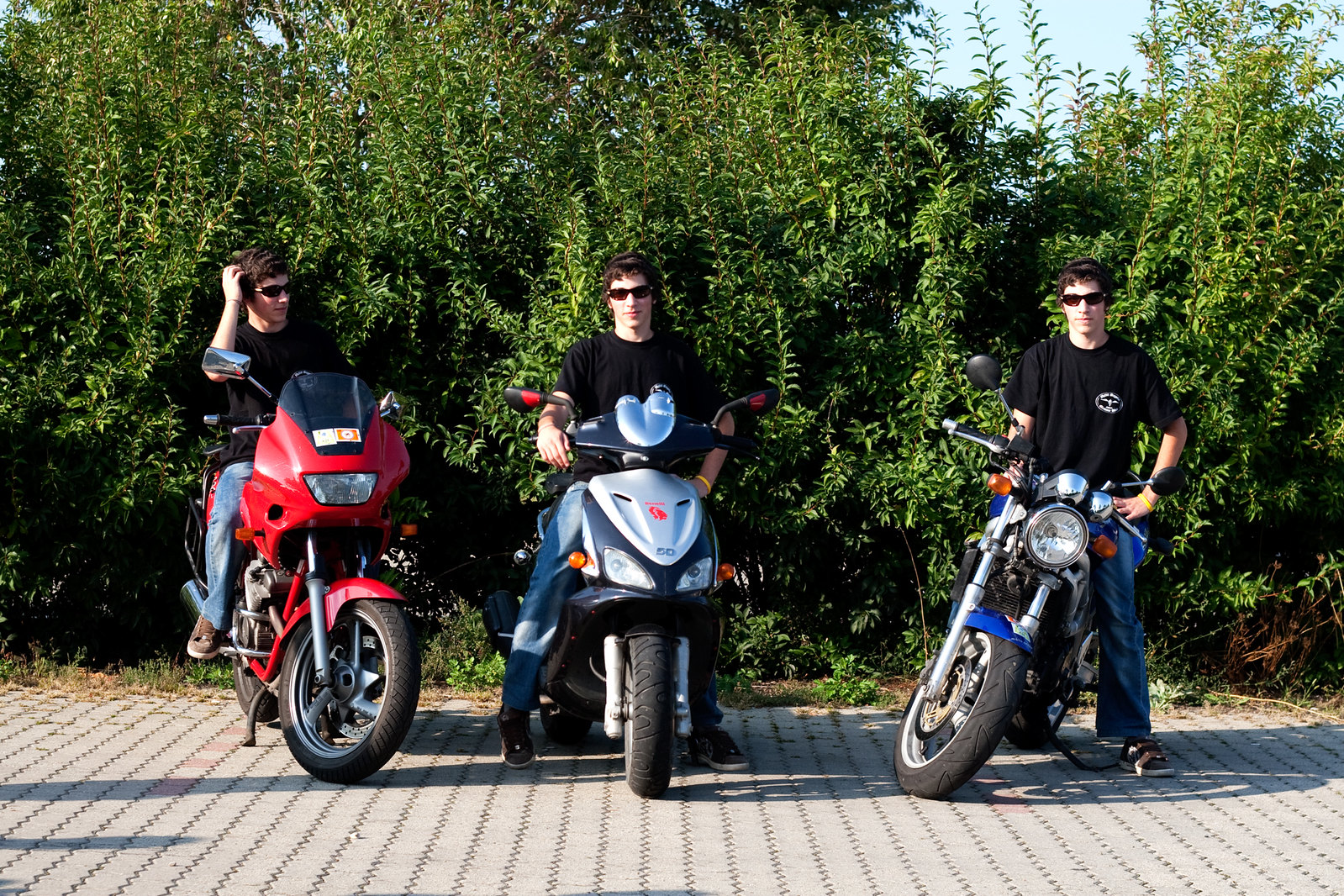This detailed photograph features three individuals astride motorcycles, lined up side by side on jagged paving stones with dense trees and bushes forming the background. Each rider is wearing a black T-shirt and brown sunglasses, and all have blue jeans with brown shoes featuring white laces. The person on the left, mounted on a red motorcycle with a prominent windshield and silver mirrors, has their right hand up, seemingly scratching their head, while their head is turned slightly to the right. The rider in the center, on what appears to be a scooter with a silver body, stands with one hand on the throttle, facing directly at the camera. Finally, the individual on the right is on a blue motorcycle, characterized by black wheels, silver handles, and twin black mirrors. This third rider stands with his left hand on his hip and is distinguished by a small white lock graphic on the left side of his T-shirt. The sky is faintly visible in the upper-right corner beyond the thick foliage.